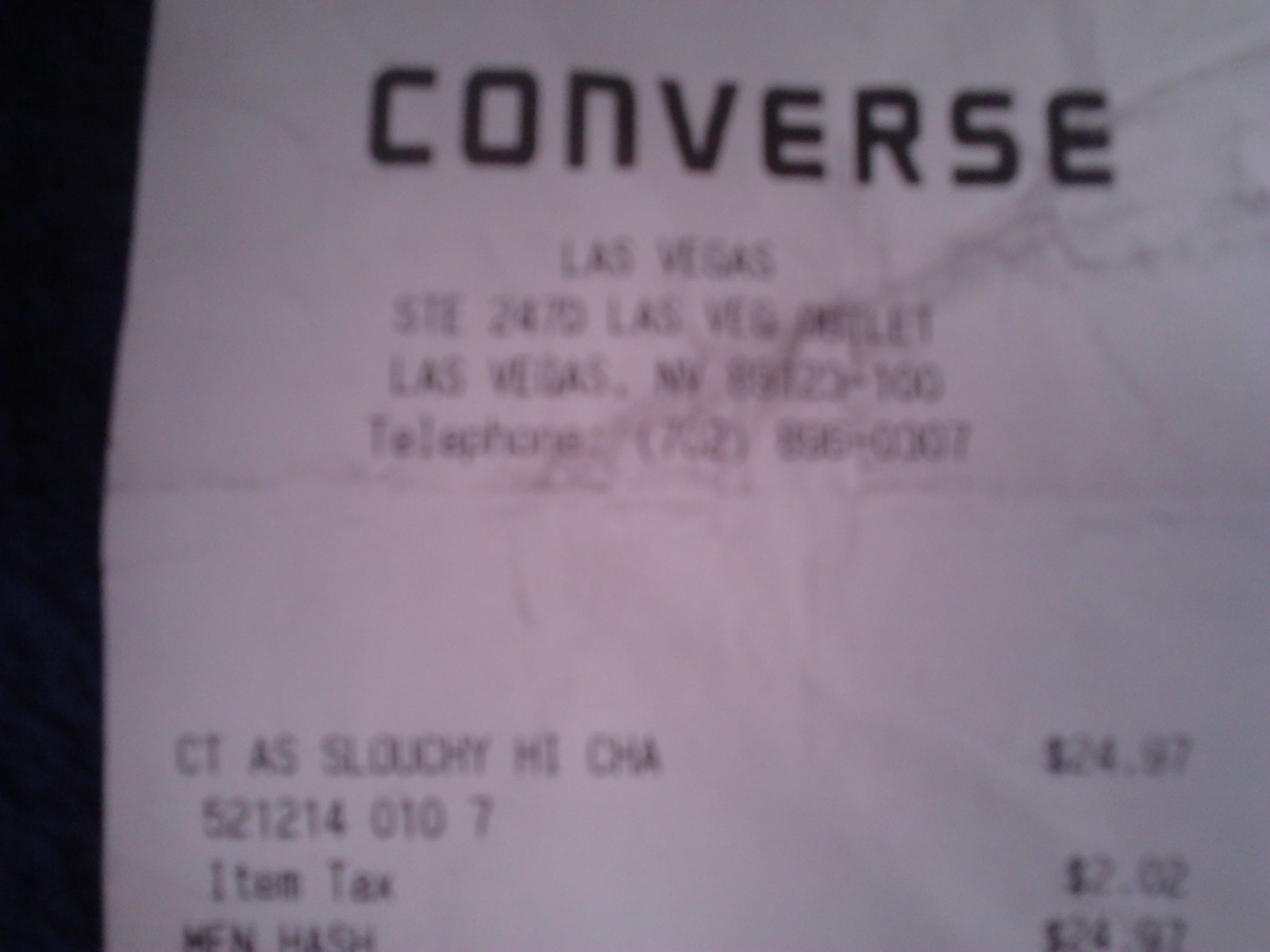Close-up photograph depicting a slightly blurry, low-resolution receipt. On the left side, a black border suggests the edge of a table. The top part of the receipt is visible, with the brand name "Converse" prominently printed at the top, followed by "Las Vegas" beneath it. Further down, though difficult to read, the text appears to indicate "S11-2470 Las Vegas Outlet" and "Las Vegas, Nevada." To the right, the price "$24.97" is clearly discernible.